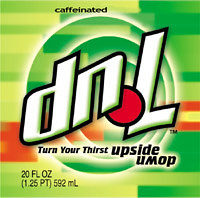This low-resolution color photo features an advertisement for a soda known as "Seven Upside Down," which appears to have been promoted in the early 2000s. The central focus is the classic 7UP logo, which is upside down, creating an effect that almost makes it look like it says "DNL." The logo consists of the number "7" and the word "UP" separated by an iconic red circle dot. Surrounding the logo are concentric circles in white, adding a layered look.

Above the upside down logo, the word "caffeinated" is prominently displayed. Beneath the logo, the phrase "Turn your thirst upside down" is written, with the word "down" itself also upside down. 

The background is composed of various shades of green, including lime green, giving it a vibrant, dynamic appearance. Additionally, there is a red stripe that runs horizontally through the middle of the design. At the bottom left corner, the advertisement specifies the serving size, saying "20 fluid ounces, 1.25 pints (592 milliliters)."